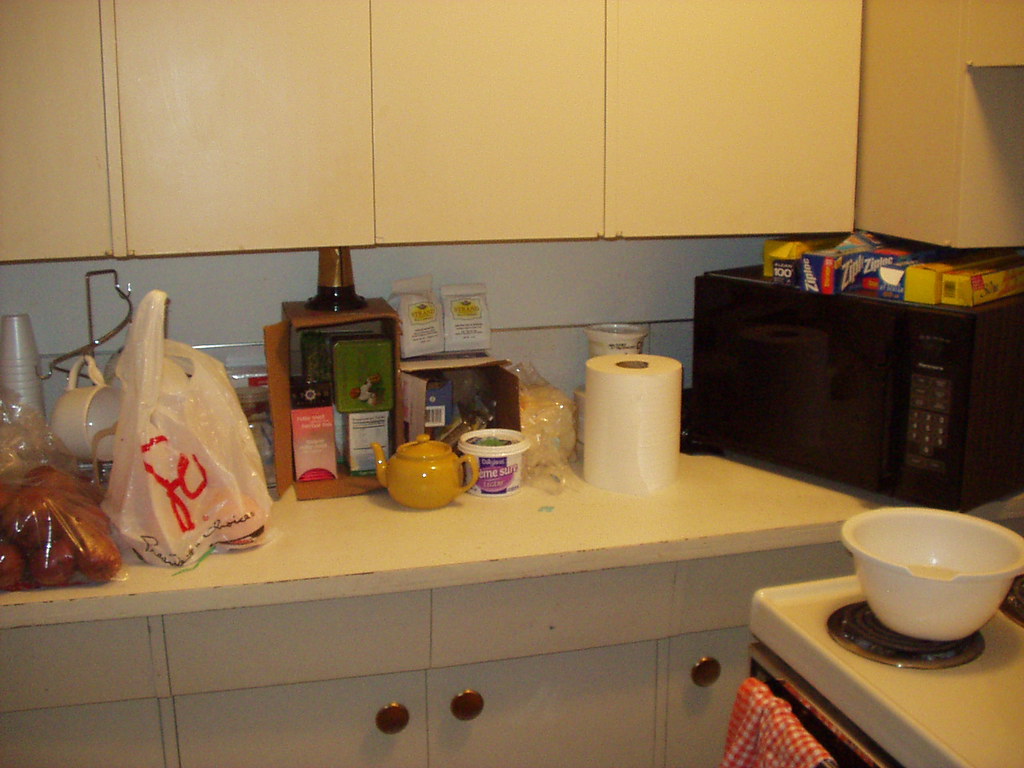This image captures a cozy and cluttered corner of a kitchen. The top portion of the scene features a set of pale yellow cabinets sans knobs, creating a minimalist yet charming look. Beneath these cabinets, a gray wall provides a muted backdrop that highlights the items on the yellow countertop below. The countertop itself is adorned with an array of miscellaneous items: a bottle that appears to be liquor, a roll of toilet paper, a small golden-yellow teapot, and other scattered objects. Below the countertop are light tan cabinets equipped with round knobs.

In the lower right corner of the image, the front left burner of a stovetop is partially visible, with an empty white bowl placed on it. Draped over the stove handle is a red and white checkered dish towel, adding a touch of homely warmth to the scene. A white grocery bag, slightly folded and seemingly filled with undetermined items, occupies part of the countertop space.

Towards the middle of the right-hand side, a black tote box is positioned, containing Ziploc bags and what appears to be the tops of yellow cereal boxes. Additionally, a white coffee cup is seen hanging from a silver hook or rack, offering a glimpse into the everyday functionality of the space. The intertwining layout presents the countertop along the left wall and the stove against an adjoining wall, forming a right angle that captures the organized chaos typical of an active kitchen.